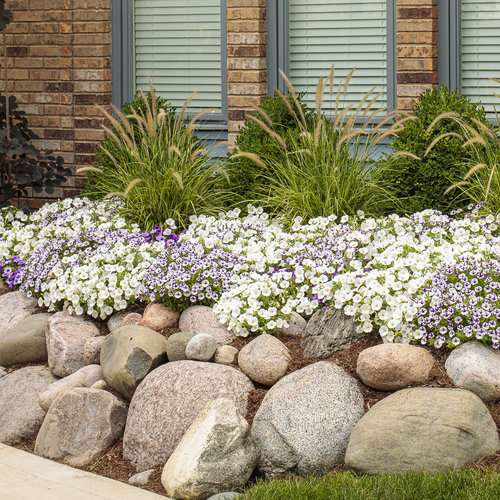This image vividly captures the front of a house with meticulous landscaping. At the bottom of the image, there's a small patch of grass on the right-hand side and a tiny sliver of the sidewalk on the left. Above the grass, a layer of large and small rocks of various colors, including gray and reddish tones, is arranged. Next, there's a strip of white and light purple flowers, likely a type of daisy, with more white flowers dominating the scene. Above these flowers, a row of bushes with long stems and fluffy tips can be seen, resembling cattails. Behind this lush greenery stands a building constructed with predominantly brown and tan bricks, interspersed with some white-tinted ones. The house features three windows with closed blinds, framed by bluish windowsills. The combination of vibrant plants and sturdy brickwork creates a charming yet ambiguous setting, whether it be residential or commercial.